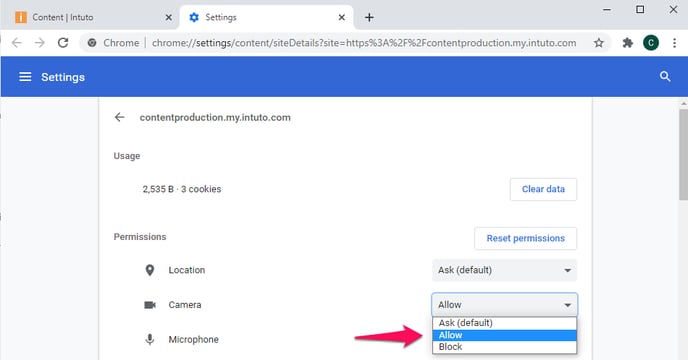This image is a screenshot of a settings page within the Google Chrome browser, specifically showing a detailed view of a website's permissions and usage information. In the browser interface, there are two tabs open. The URL bar at the top displays the address "contentproduction.my.intudo.com".

Below the URL bar is Chrome's settings interface, marked by a prominent blue bar that stretches horizontally. On the left side of this blue bar is the 'Settings' button, while the right side features a 'Search' button.

The main content area beneath the blue bar is predominantly white and centered. At the top of this section, there is a navigation breadcrumb indicating the current site, "contentproduction.my.intudo.com," along with a back button to the left of the text. Directly below this, the page displays the data usage information "Usage: 2,535 bytes" and "3 cookies". On the right side of this section, there is a "Clear data" button, designed in white with blue text.

The subsequent section of the settings page is dedicated to site permissions. Featured here is a list of configurable settings such as Location, Camera, and Microphone. Each permission entry includes drop-down menus that offer various options like ‘Ask (default)’ and ‘Allow,’ allowing the user to specify site-specific behavior for each type of permission.